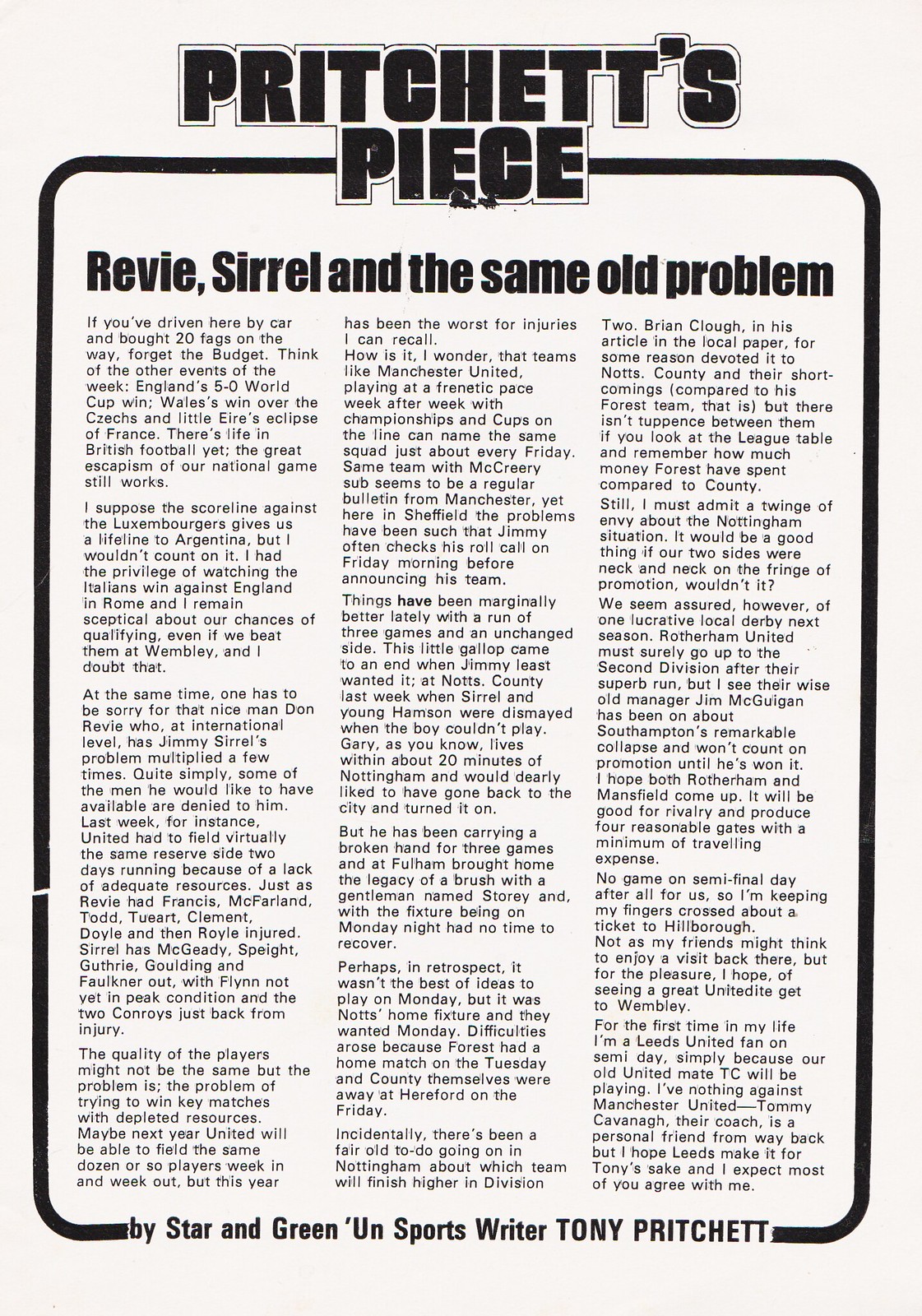This black-and-white image depicts a faded and slightly torn page from an old magazine or newspaper, featuring a detailed sports article titled "Pritchett's Piece." The article, authored by sports writer Tony Pritchett, is centered on a soccer-related discussion and spans three columns of text, formatted in a Times New Roman-like font. The main headline, highlighted in bold black lettering, reads "Revy, Cyril, and the Same Old Problem," with the subtitle "by star and green, Unsportswriter Tony Pritchett" positioned underneath it. The text covers various events and issues in British football, including England's World Cup performance, the challenges faced by managers Don Revy and Jimmy Cyril due to injured players, and the broader context of team resources and competition. The article also touches on local rivalries and the aspirations for team promotions within the football leagues.